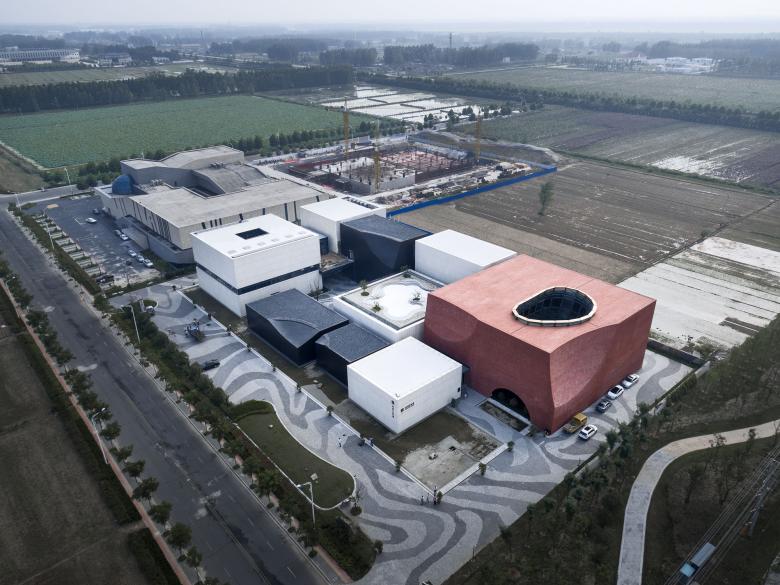This overhead, daytime aerial shot captures a building complex situated within an agricultural region. The complex comprises various cube-shaped buildings in different colors, including white, black, and a prominent red building with a noticeable hole in its roof. A larger gray, multi-story industrial building also stands out. Surrounding this facility, there are both agricultural fields and patches of greenery. To the left, a road runs diagonally from the bottom to the upper left of the image, flanked by fields. The background features a blend of tall trees and additional buildings, suggesting a mix of residential and industrial areas. The skyline appears hazy, adding a soft, foggy atmosphere to the scene. Parking lots with distinctive grey and white striped patterns are visible within the complex, enhancing its industrial feel.